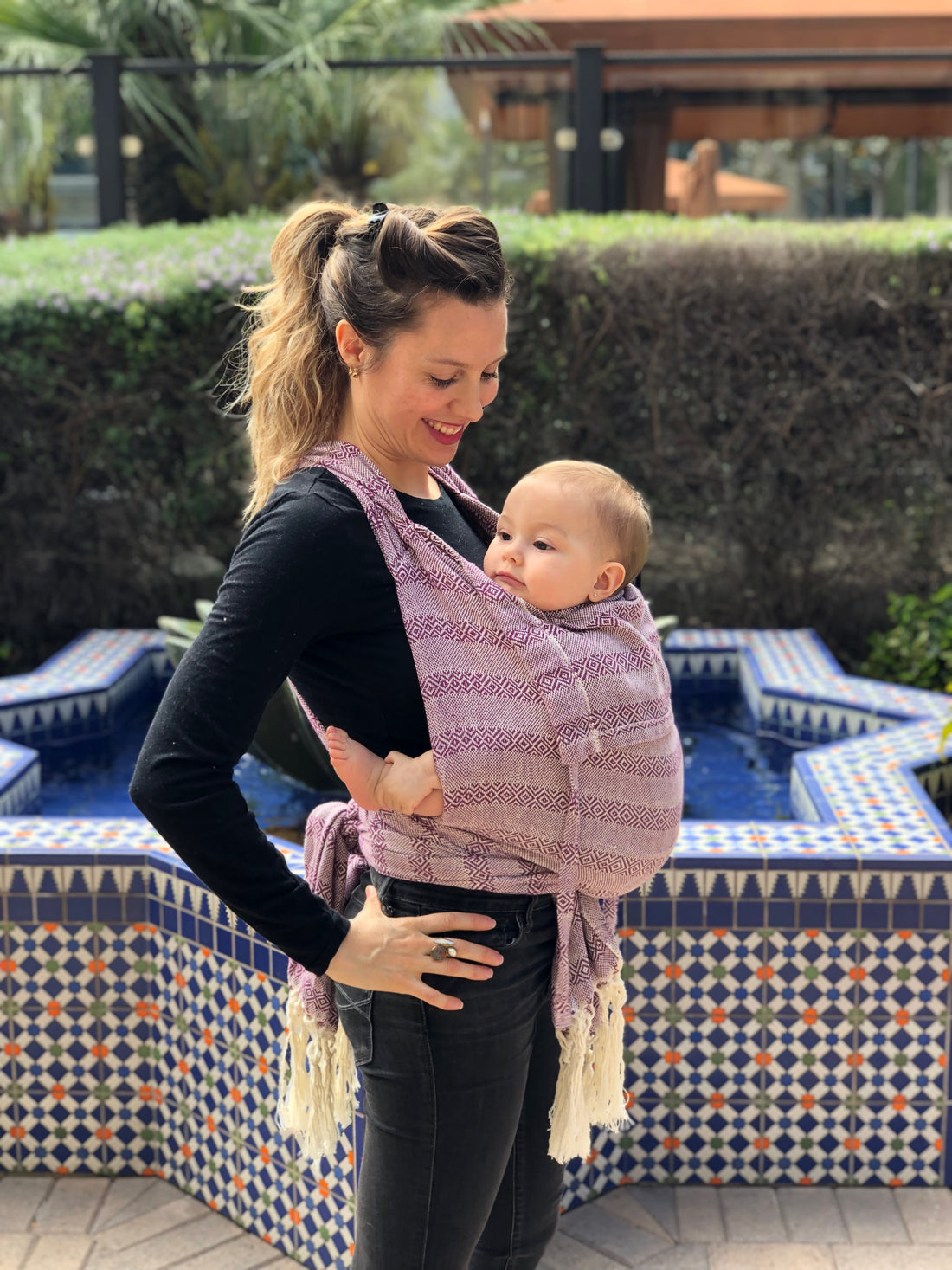In this outdoor image, a young Caucasian woman, presumably a mother, is standing in front of a small, star-shaped pool or fountain adorned with fine blue, white, orange, and green tiles. The pool features a unique star-like pattern with multiple edges. Behind the pool is a neatly trimmed hedge that runs parallel like a fence, beyond which some trees and an indistinct brown wooden structure are visible. The woman has dark brown hair with blonde highlights, styled in a ponytail with a decorative twist at the front where her bangs are. She is dressed in a long black top and black jeans, with her hand resting on her hip as she smiles down at the baby she is carrying. The baby, nestled in a cloth sling wrapped around the woman's shoulders and waist, has short brownish hair and a sweet expression, gazing to the left while clutching its own feet. The mother exudes warmth and tenderness, enhancing the serene and picturesque setting.